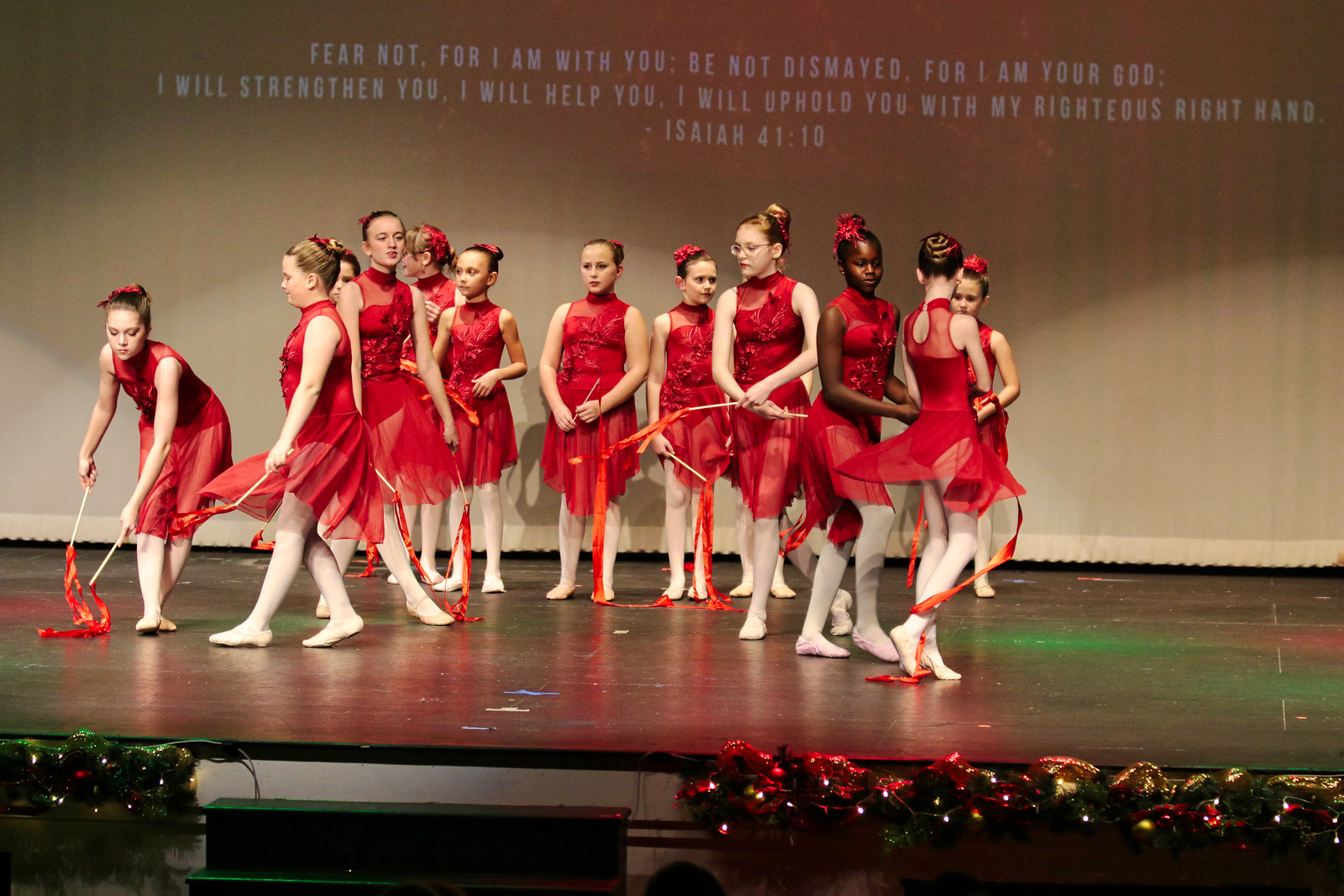A group of 12 young girls stands on a stage, all dressed in ornate red dresses with flowing tulle skirts and white tights. Each girl’s hair is styled in a bun adorned with a red bow. They hold batons with bright red ribbons, matching their dresses. The formation includes four girls standing at the back facing forward and six others spread out on either side in various stages of movement, suggesting a dance performance. The stage is decorated with Christmas-themed decor, adding to the festive atmosphere. Above the girls, a PowerPoint slide features the Bible verse, "Fear not, for I am with you. Be not dismayed, for I am your God. I will strengthen you. I will help you. I will uphold you with my righteous right hand. Isaiah 41:10." The setting appears to be indoors, possibly within a church, during a performance event.